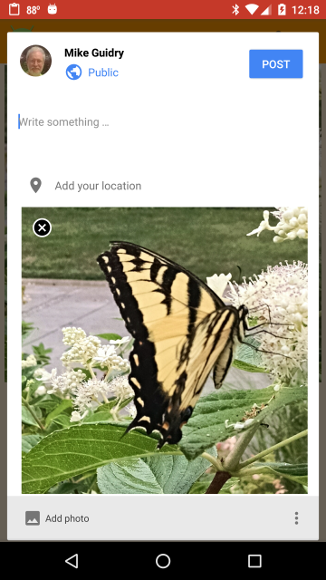This smartphone screenshot captures a Facebook post creation screen. At the center of the pop-up box, displayed against a white background, is a square photograph of a yellow and black butterfly resembling a monarch, perched delicately on a stalk with green leaves and dotted with small white flowers.

The post is authored by a man named Mike Guidry, whose name appears in the upper left-hand corner alongside his profile picture. Just below his name is a blue globe icon labeled "Public," indicating the post's visibility. To the top right corner of this pop-up, there is a blue "Post" button with white text. A vertical blue cursor line is situated under Mike Guidry's name within a text box that prompts "Write something..." Additionally, there is a small "Add your location" prompt at the top left-hand side of the image. Directly beneath this section, on a gray banner, there is an "Add Photo" option.

The top of the image features a red banner displaying the current temperature of 88 degrees and the time, 12:18 PM. At the lower part of the screenshot, there is a black banner hosting three icons, presumably representing navigation options on the smartphone.